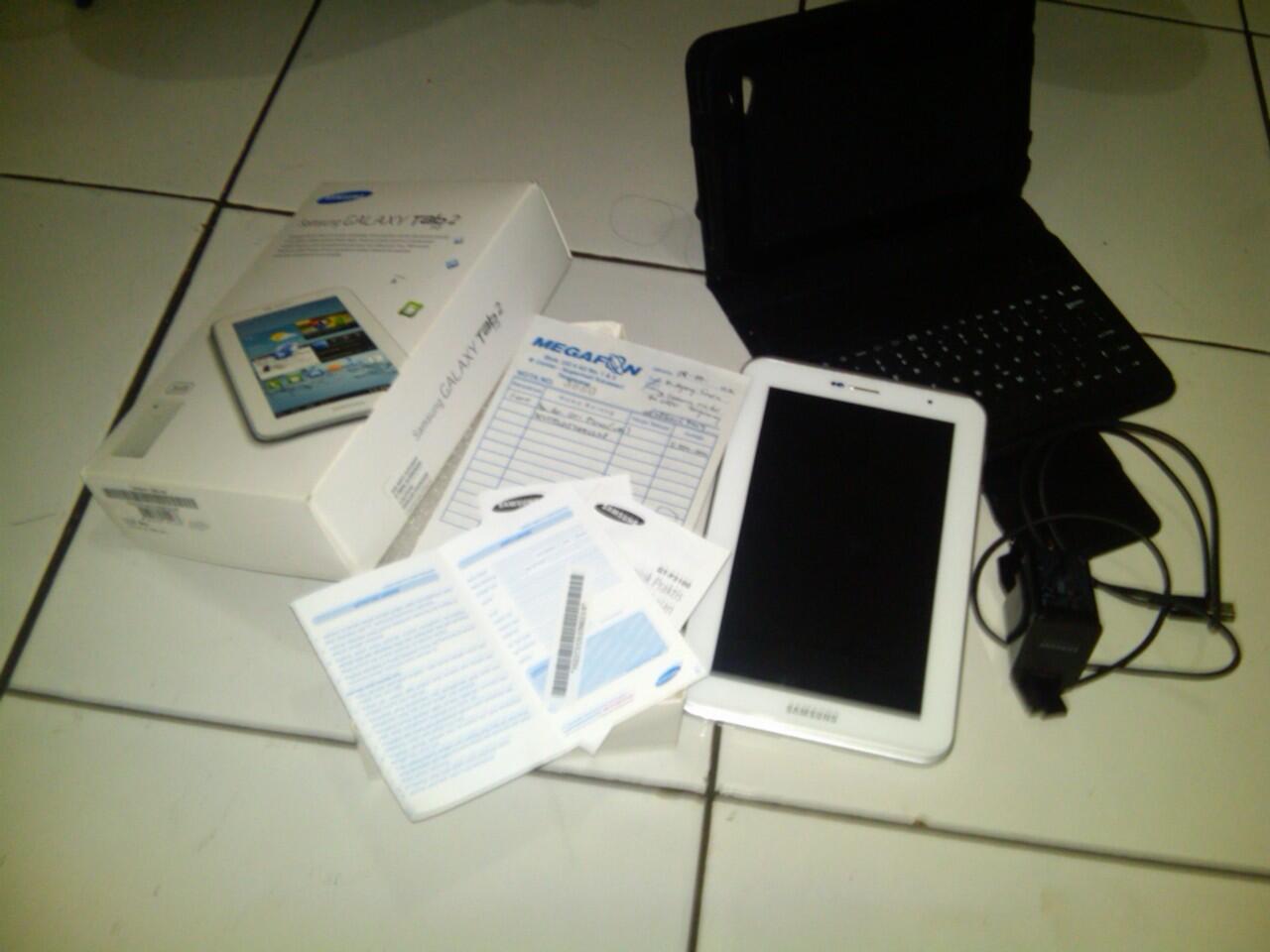The image depicts a cluster of electronic devices and accessories arranged on a white tiled floor. Central to the image is a white Samsung Galaxy Tab 2 tablet, approximately 7 inches in size, accompanied by its partially opened box and instruction manuals. Positioned to the right of the tablet is a small black laptop, which lies open but is powered off, with its charger resting nearby. Additional items, including what appear to be receipts and booklets related to the tablet, are scattered to the left of the main setup. The placement of the objects is both horizontal and vertical, creating a somewhat organized yet casual arrangement, suggesting an indoor setting. The color scheme of the items features predominantly white, black, and accents of blue on the lettering of the tablet's box.